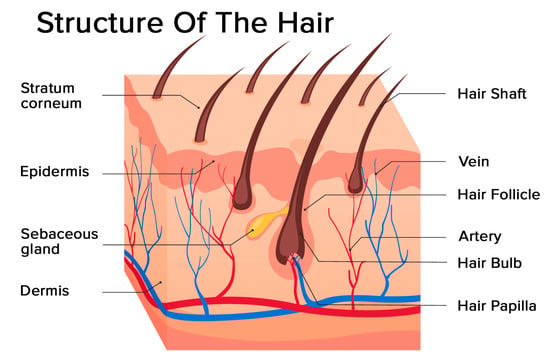This is a detailed textbook diagram titled "Structure of the Hair," illustrating the various layers of the skin and hair components. The center of the image features a flesh-colored, predominantly pinkish cube from which several hairs emerge. These hairs, brown in color, start thick at the base and taper off towards the end, angling towards the right. The diagram marks the different layers and associated structures: at the base, we see the dermis layer including the hair bulb and hair papilla, which is crucial as the root of the hair. Surrounding these are red and blue veins and arteries, indicating blood flow. The sebaceous glands, sources of potential acne, are also present in this layer. Above the dermis is the epidermis, where some veins persist, and at the very top is the stratum corneum, the outer visible layer of skin, accompanied by the protruding hair shaft. The diagram is meticulously labeled: on the left side, the labels read from top to bottom—stratum corneum, epidermis, sebaceous gland, and dermis. On the right side, the labels include hair shaft, vein, hair follicle, artery, hair bulb, and hair papilla, each pointing to their respective locations in the image.